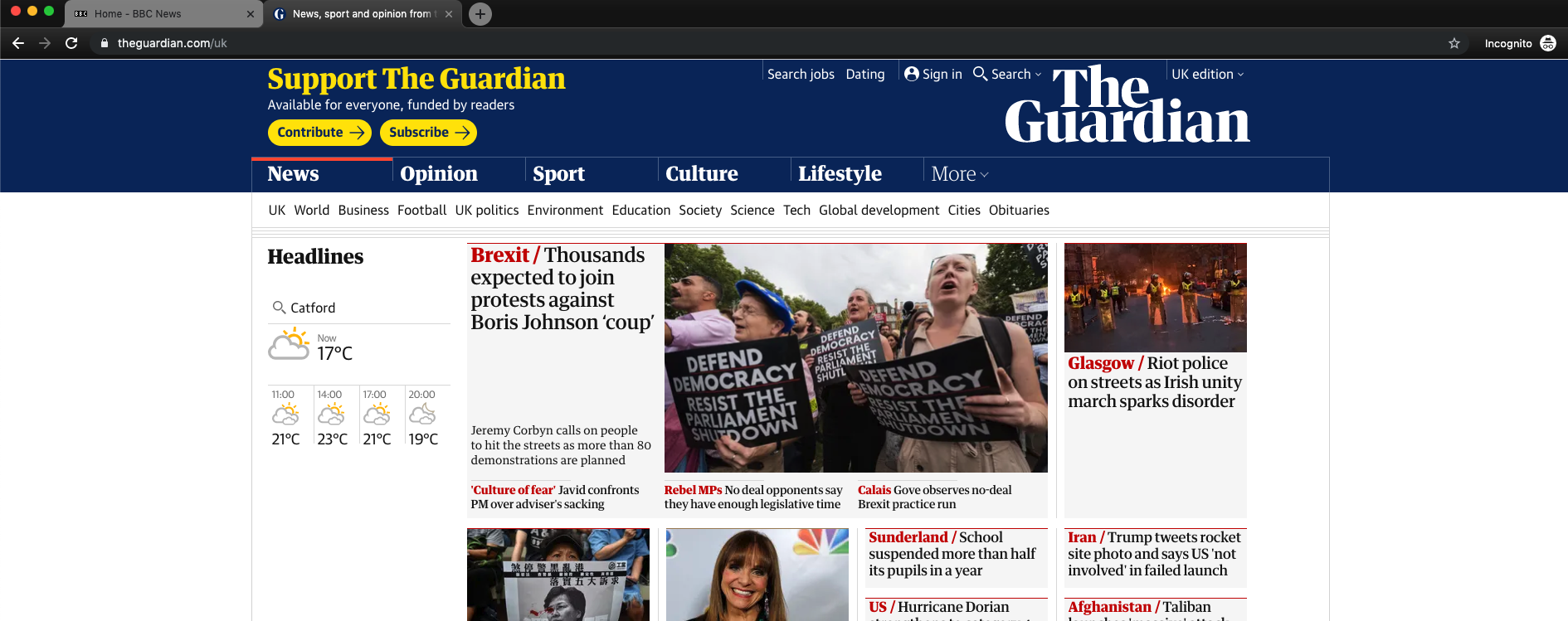The image is a screenshot of the homepage of The Guardian's UK website, visible at the URL "theguardian.com/uk." The website features a prominent banner at the upper left corner urging visitors to "Support The Guardian." This banner is notable for its yellow text on a navy blue rectangle background and includes the subtext "Available for everyone, funded by readers" in white. Below this message are two yellow buttons labeled "Contribute" and "Subscribe."

At the top navigation bar, the site offers links for "Search jobs," "Dating," "Sign in," "Search," and "UK Edition." The title "The Guardian" is prominently displayed towards the right side of the screen. Beneath this, primary navigation tabs include "News," "Opinion," "Sport," "Culture," "Lifestyle," and a dropdown for "More."

Further down, there are sectional headers for various news categories: "UK," "World," "Business," "Football," “UK Politics,” "Environment," "Education," "Society," "Science," "Tech," "Global Development," "Cities," and "Obituaries." The right side of the page contains weather information, while the main body showcases an array of news articles accompanied by relevant images.